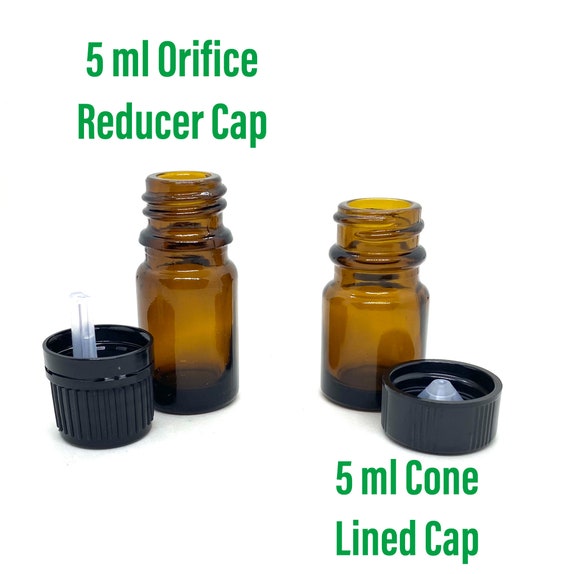The image depicts two empty amber glass bottles with their caps off, set against a stark white background. Green text provides descriptions for each bottle. The bottle on the left is taller and narrower with green text above it reading "5 milliliters orifice reducer cap." Next to it lies its cap, which is a tall black one with a clear plastic orifice reducer inside, consisting of one or two cylindrical pieces. The bottle on the right is shorter and wider with green text beneath it stating "5 milliliters cone-lined cap." Its corresponding cap, also black but shorter, has a visible clear plastic cone inside. The bottles, caps, and their reflections are the only elements in this minimalist and informative composition.